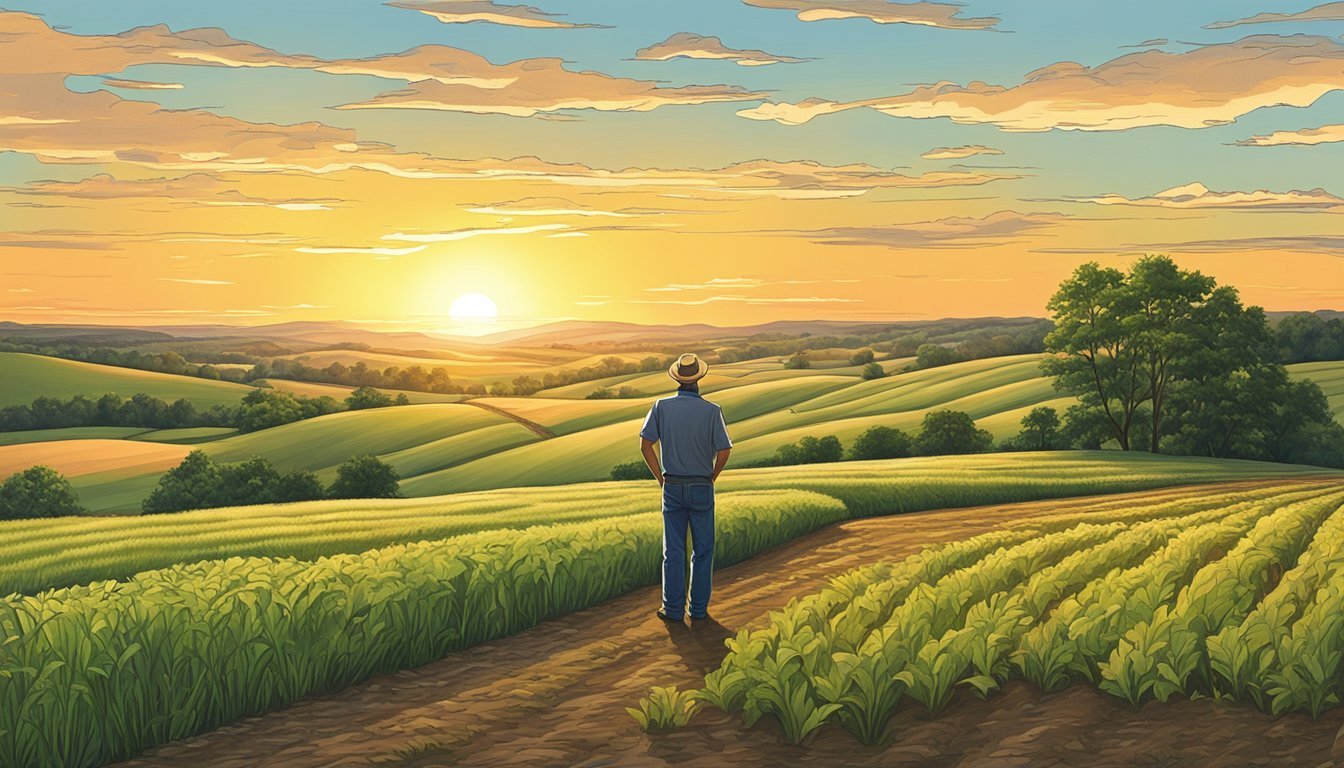The painting is a serene and detailed country scene showcasing rolling hills and cultivated farmland under a vibrant sunset sky. Dominating the foreground are rows of light green crops, possibly soybeans, growing in neat parallel lines alongside a dirt path. A farmer, dressed in blue jeans, a short-sleeved blue shirt, and a tan cowboy hat, stands on this path with his hands in his pockets, facing away from the viewer. The serene landscape stretches out behind him, featuring grassy hills dotted with a few trees, one notably larger than the rest, and dark green shrubs forming a quilt-like patchwork over the terrain. In the background, the horizon is set aglow with an orangey-yellow sunset that merges into a partly blue sky accented by fluffy clouds. The distant mountains, painted in hues of purple, add depth and tranquility to the scene, making it a beautifully peaceful and picturesque illustration.